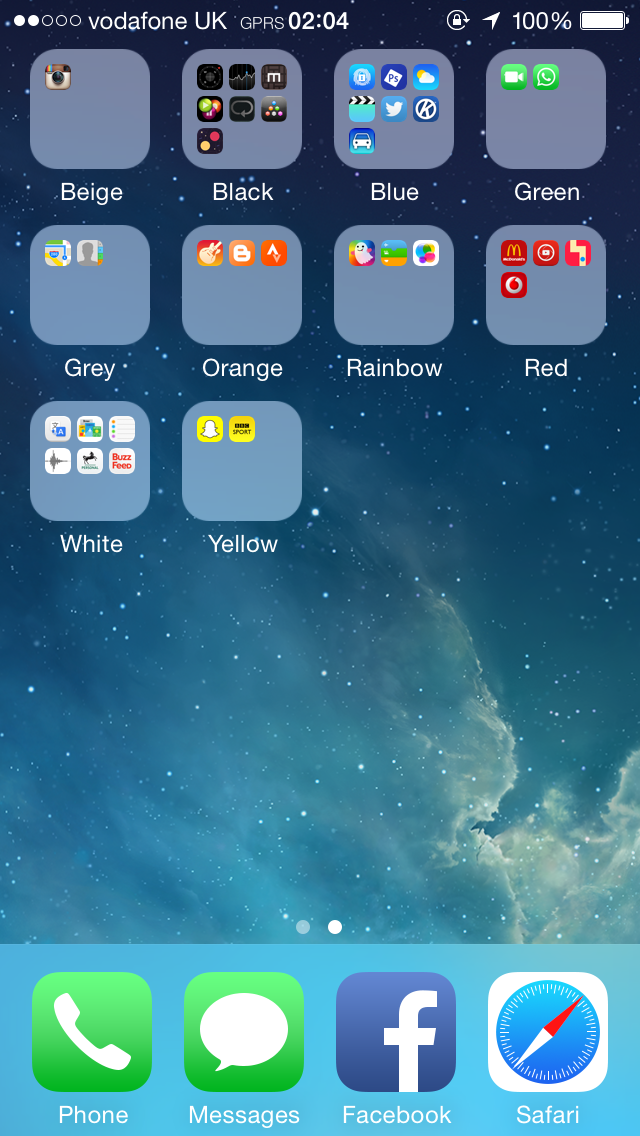This vertically oriented image depicts the home screen of an iPhone with a backdrop of a starry, cloudy night sky, featuring rays of light emanating from the bottom-right corner. The bottom dock of the screen hosts four frequently used apps: Phone, Messages, Facebook, and Safari, arranged from left to right.

Along the top of the screen, the status bar indicates the device is connected to Vodafone UK with a signal strength of two bars. A GPRS logo is visible, denoting the data connection type. The current time, displayed centrally in this bar, is 2:04. To the right of the time, a series of icons is present, including a lock symbol, an arrow, and a battery indicator showing a full charge at 100%, represented both numerically and visually.

The home screen features ten organized folders filled with various apps, meticulously arranged as follows:

- The top row consists of folders named Black, Blue, Black, and Green.
- The second row includes folders labeled Gray, Orange, Rainbow, and Red.
- The bottom row contains the last two folders named White and Yellow.

Overall, the image provides a clear and organized view of the iPhone's home screen setup, set against a serene, celestial background.